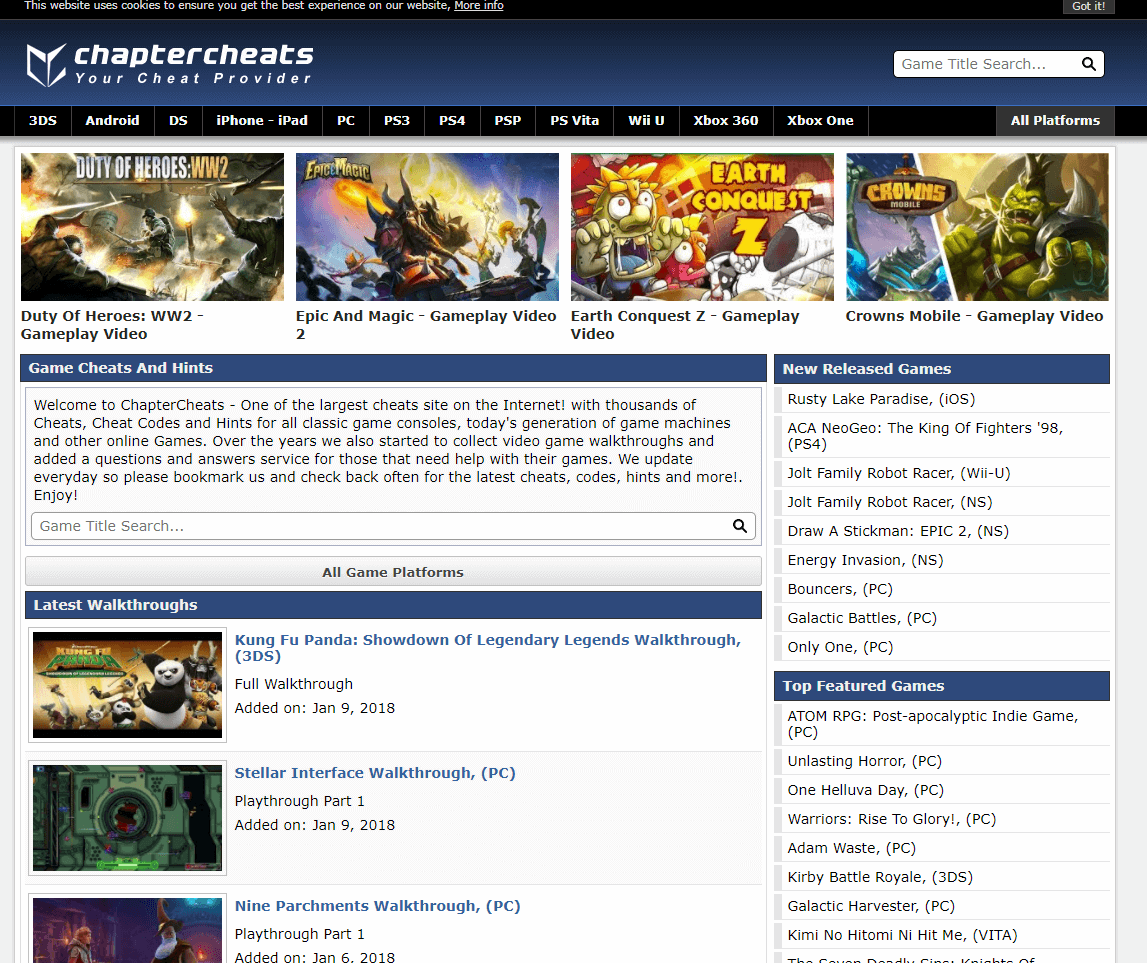"Discover a treasure trove of gaming secrets on Chapter Cheats, one of the largest and most comprehensive cheat code websites on the internet. This nostalgic platform, reminiscent of early 2000s web design, offers thousands of cheats and cheat codes for a myriad of video games, including popular titles like Duty of Heroes and Epic Magic. Stay ahead of the game with the latest releases and featured games, all in one place. Whether you are a seasoned gamer or a newcomer looking to unlock hidden features, Chapter Cheats is your go-to source for all gaming cheats and tips. Find your ultimate cheat codes here at Chapter Cheats, your trusted cheat provider."